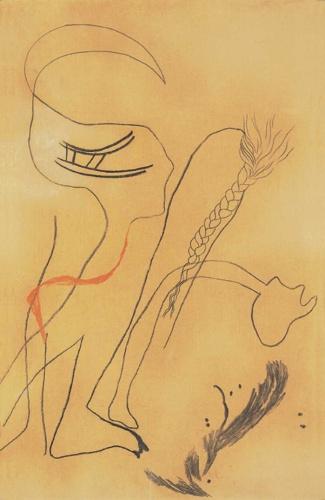This is a vertically aligned rectangular drawing in portrait orientation, known as "Braids or Braided Hair Composition" by Lahos Vajda, created in 1939. The background is a blend of brown tones, mostly medium brown with some areas of light brown, resembling a parchment color. The artwork, appearing childlike and simplistic, features abstract shapes rendered in crayon or pencil, primarily in orange, black, and gray hues. 

At the top left, a red curved line outlines a shape that could suggest a nose and a chin, descending into a foot-like form. To the right of this, an intricate design resembling braided hair or a twisted rope extends downward, composed of black, swirling lines. There is also an orange ribbon-like scribble and several black and gray scribbles across the composition.

The central figure appears cucumber-like with hairy black lines at the top. Below it, one can perceive a giraffe's neck shape with a black feather curling beneath. The artwork is a modernist surrealist piece, filled with abstract shapes that elicit a sense of imaginative ambiguity.